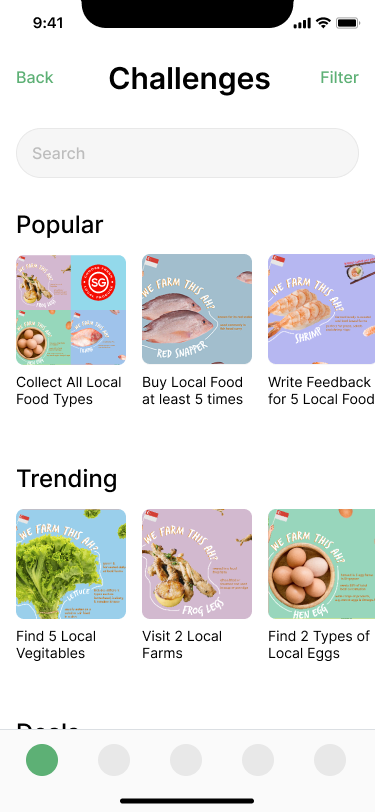The image depicts a user interface for a food filter application. At the top, there is a green button labeled "Back," followed by a middle section with bold black text reading "Challenges." To the right of this, in green text, it states "Filter." Below this, there is a search bar with a placeholder text that says "Search."

Underneath the search bar, a heading labeled "Popular" is displayed, followed by three segments:

1. The first segment states "Collect All Local Food Types" and features a four-by-four grid with various food items.
2. The second segment reads "Buy Local Food at Least Five Times," accompanied by an image of fish and text saying "We Farm This Red Snapper."
3. The third segment entails "Write Feedback for Five Local Foods," featuring an image containing shrimp and a person using chopsticks with a sushi roll.

Further down, a heading labeled "Trending" is shown, which is followed by another set of three segments:

1. The first of these segments says "Find Five Local Vegetables," illustrated with a picture of lettuce and text that partially says "We Farm This R…"
2. The second segment instructs to "Visit Two Local Farms," with an image of grilled frog legs and text stating "We Farm This Frog Legs."
3. The third segment advises to "Find Two Types of Local Eggs," including a picture of a bowl with eggs and text reading "We Farm This Hen Egg."

This caption provides a comprehensive overview of the interface elements and their respective descriptions.